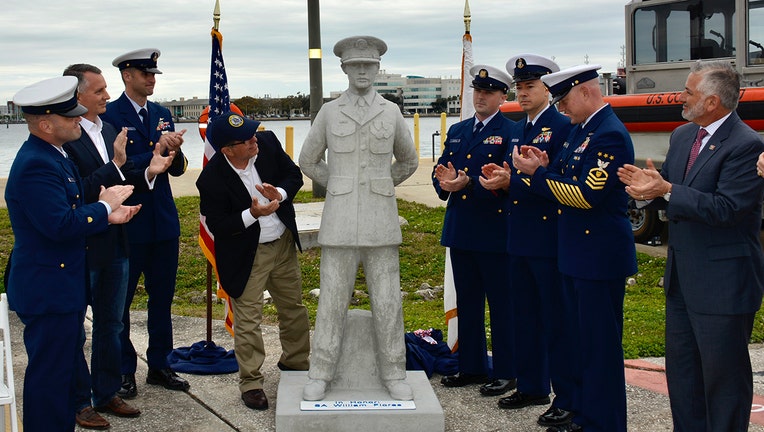This photograph captures a commemorative ceremony featuring a semicircle of individuals around a gray statue of a uniformed military figure, likely a World War II Coast Guard officer, with a plaque at its base. Among the attendees, there are six U.S. Coast Guard personnel in blue uniforms and sailor caps. The right side of the statue is flanked by three Coast Guard members, followed by a man in a suit, while the left side has two more Coast Guard personnel. A man in a blazer, khaki pants, and a baseball cap with a government logo leans forward, closely inspecting the statue's face. Two additional gentlemen in suits stand on either side, with all of them appearing to applaud. An American flag is positioned behind the attendees, along with a body of water and a Coast Guard boat in the background. A patch of grass and a cloudy, slate-blue sky complete the scene, with a distant city skyline visible.